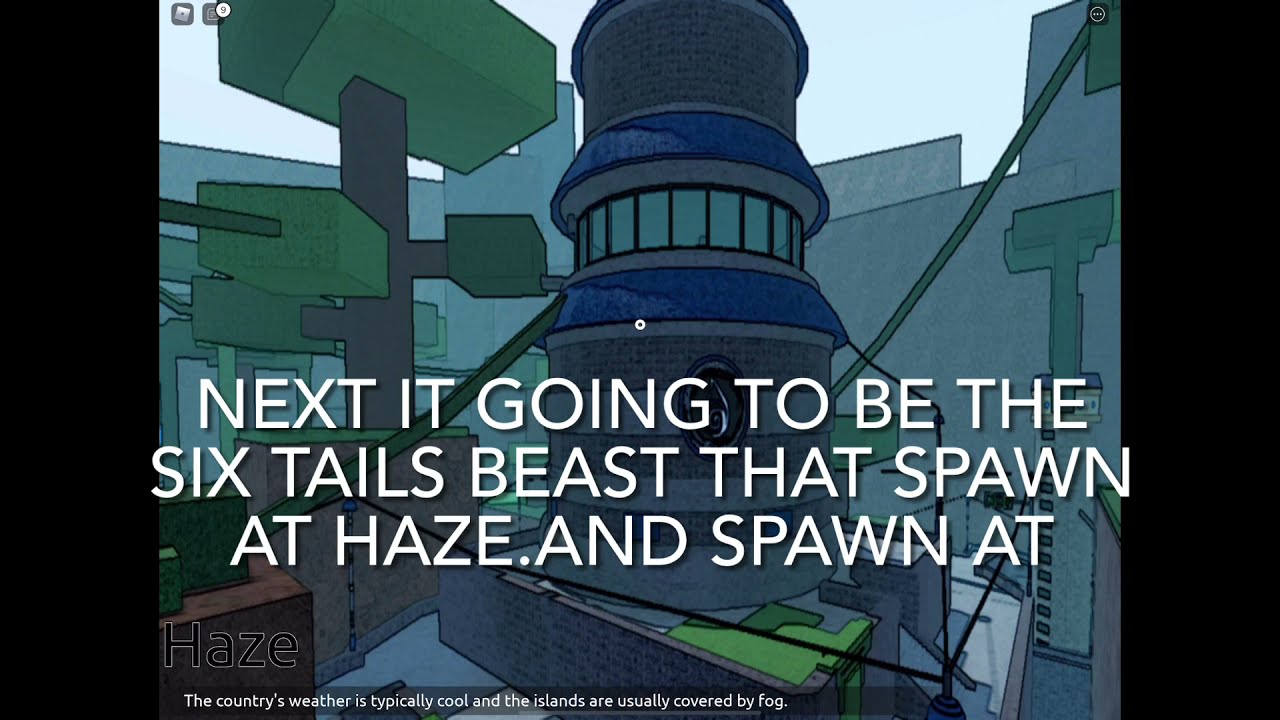The image is an animated illustration of a complex structure, primarily in shades of blue and green. It features a central cylindrical tower with windows that wrap around its middle section. The tower appears to be divided into several tiers, and it's constructed from what looks like bricks with blue siding. Emerging from either side of the tower, there are long, thin dark green tubes or rectangular prisms. To the left of the tower stands another gray structure resembling a tree with green square attachments along its branches, and various green rectangular prisms protrude from the holes in this structure. A gray backdrop frames the tower and the tree-like structure, enhancing their prominence. 

The image includes text elements: in large white letters near the bottom center, it reads, "Next, it going to be the six tails beast that spawn at Haze and spawn at." Additionally, towards the lower left corner, the black-outlined word "Haze" appears. Below it, in tiny white letters, it states, "The country's weather is typically cool and the islands are usually covered by fog." Both the left and right sides of the image have black vertical rectangles, contributing to the frame of the scene.